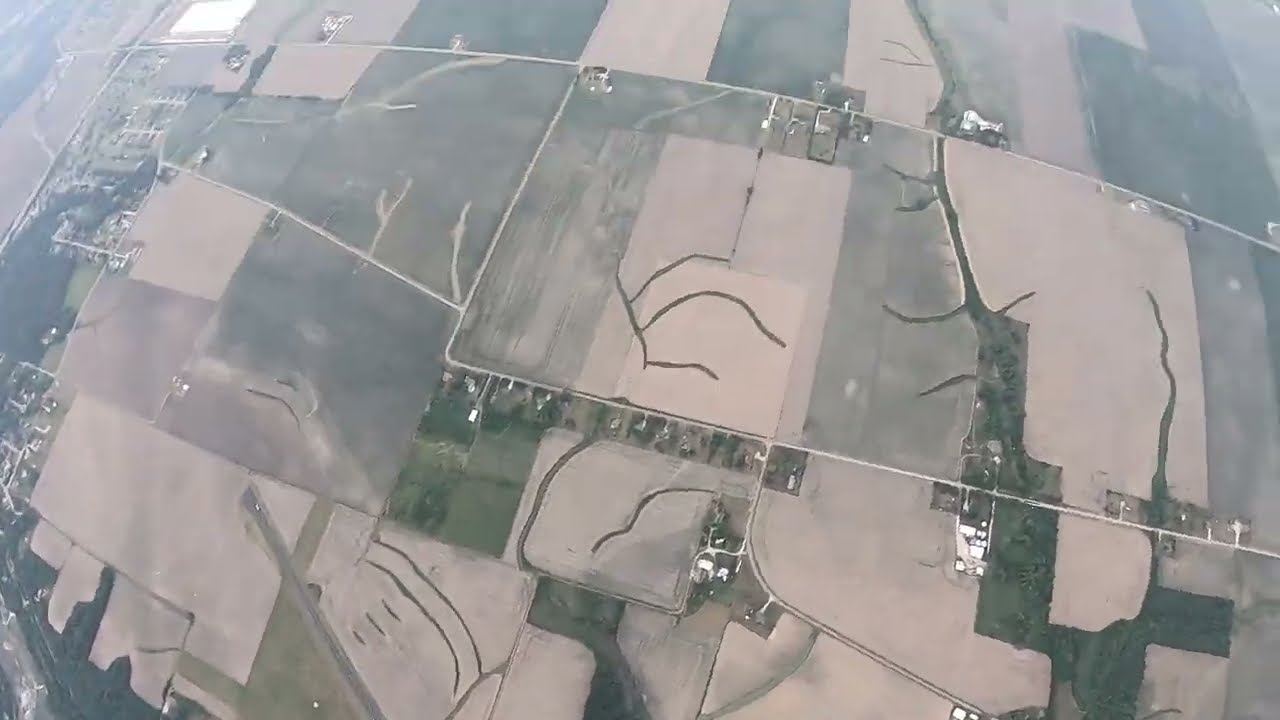The photograph captures an aerial view of a rural landscape, likely taken from a drone or during a skydiving session. The image offers a first-person perspective, looking down at a vast patchwork of farmland. These fields are neatly divided into squares and rectangles, bordered by roads, creating a structured grid layout. Predominantly, the fields display various shades of green and brown, from light earthy tones to darker hues, indicating different stages of crop growth or types of vegetation. Snaking through some of these fields are narrow waterways or irrigation channels, adding a dynamic element to the otherwise geometric expanse. 

On the left side of the image, a small suburban development with scattered houses and a few larger buildings can be seen, though their diminutive size underscores the high vantage point of the photograph. Trees interspersed among the plots and structures add a touch of natural variety to the scene. Overall, the landscape depicted is predominantly agrarian, with meticulously divided sections of land showcasing different uses and stages of cultivation.